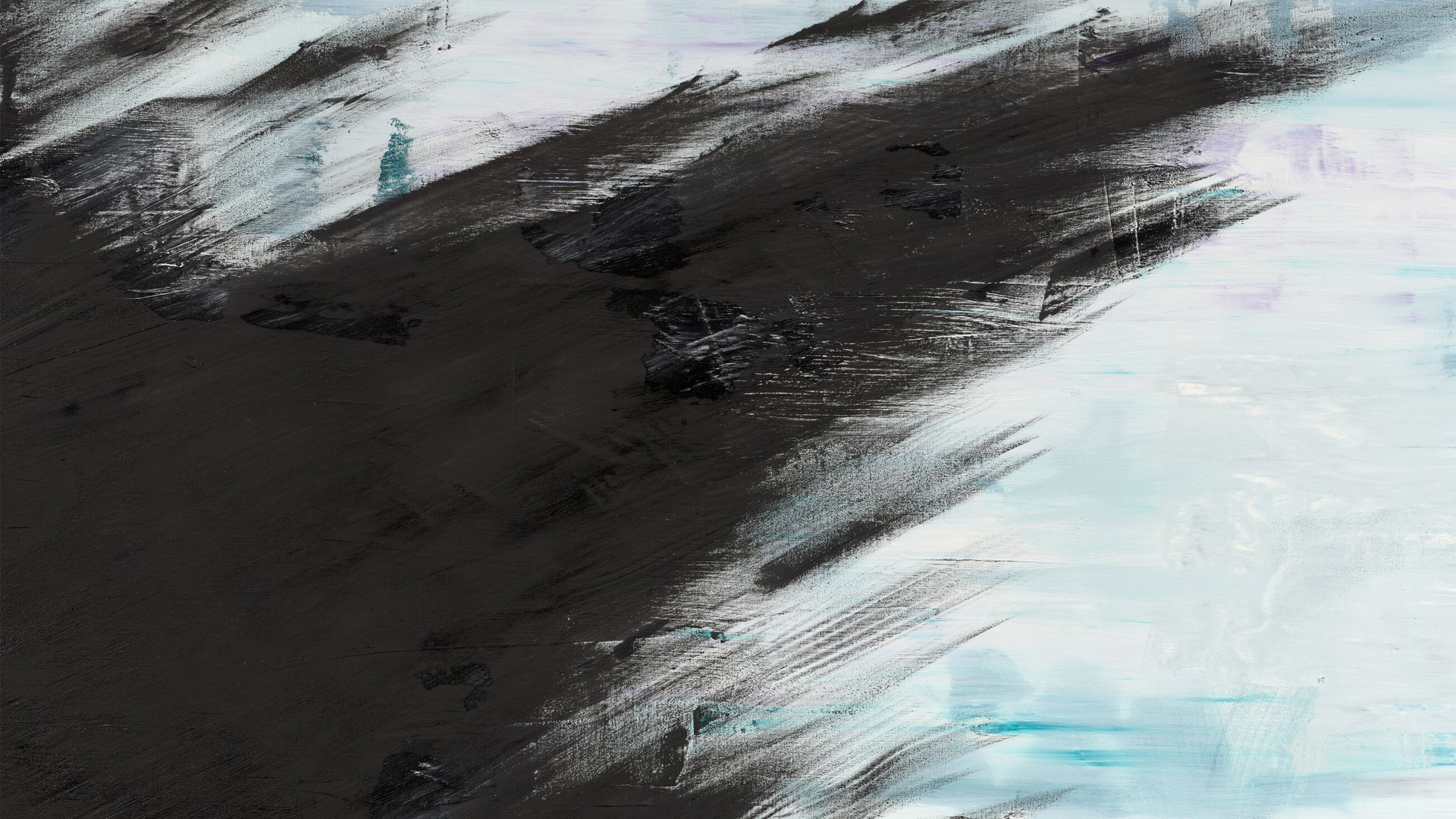This rectangular abstract painting predominantly features black, dark gray, white, and blue with hints of purple. The composition is dominated by a large, shadowy black section stretching from the lower left to the upper right corner, blending into softer shades as it transitions. In the middle of this black area, there's an indistinct object, surrounded by a stark contrast of colors. Above the black section, a white area hosts a tiny, dark blue silhouette resembling an animal shape. Below, to the right, the painting opens up into a scene that evokes the sensation of fluffy white clouds with blue highlights and subtle purple mountains in the background. The colors blend seamlessly with no hard lines, giving the piece a smooth and flowing feel, typical of acrylic or oil techniques. The painter's strokes are visible, particularly where the white and blue hues intermix with smudges of purple and the intense black fades, illustrating a dynamic, yet harmonious transition across the canvas.